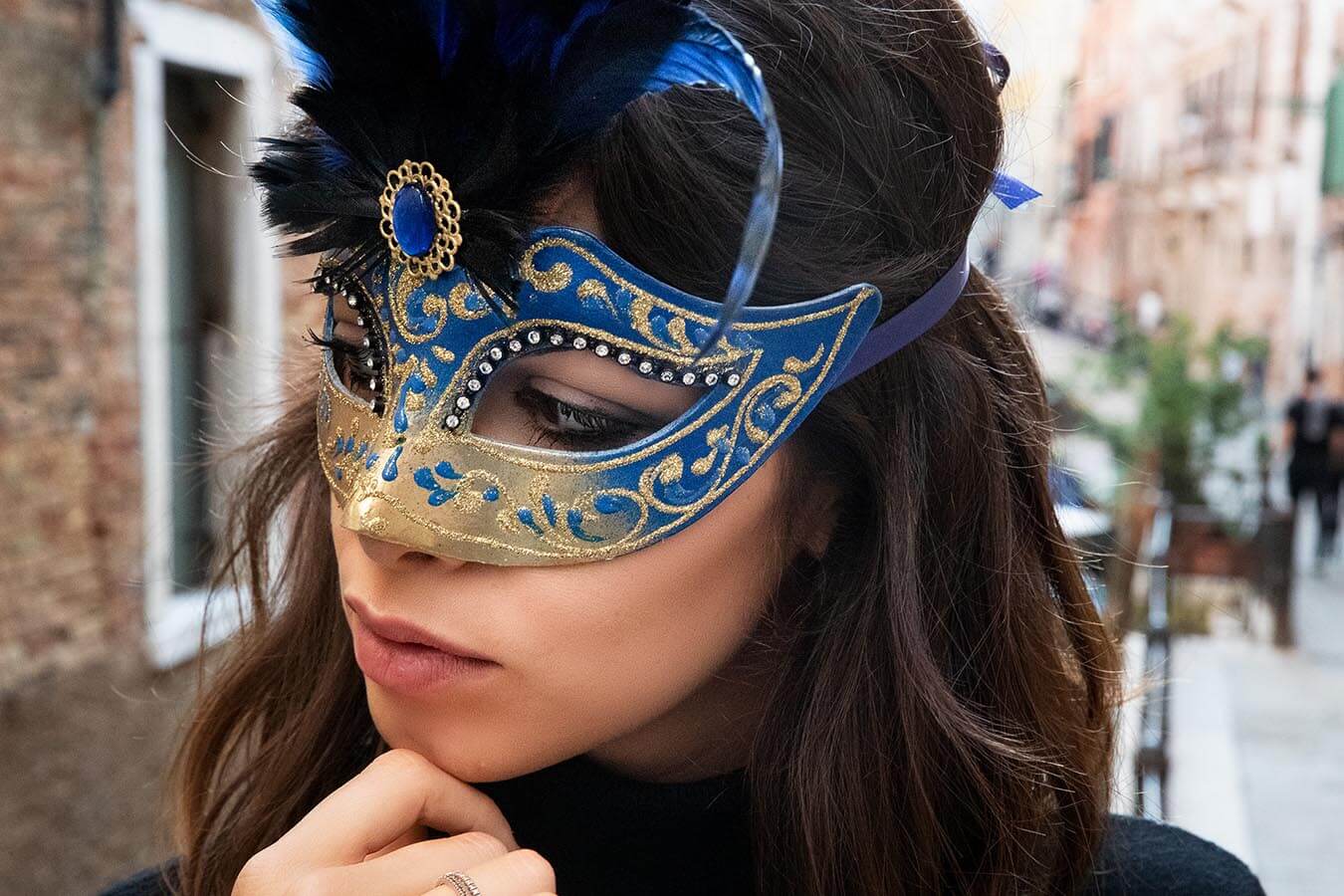A vivid and detailed close-up photograph captures a woman standing slightly turned to the left, set against a blurred street background, possibly from a European city or New Orleans. The background reveals indistinct figures and buildings, including a brick wall with a white wooden-framed window to her left. The woman has shoulder-length dark brown hair and is wearing a black top. Her facial features are finely detailed, with pronounced eyelashes and pink lips. She is elegantly propping her chin with her hand, her index finger visible. Covering her eyes, she wears an ornate blue and gold masquerade mask. The mask features intricate filigree designs with blue and gold patterns, gold glitter, and dark blue feathers held by a golden ornament adorned with a blue jewel. The mask's colors transition from blue on the outer portions to gold near the nose, creating a captivating visual effect that enhances the mysterious and celebratory aura of the image.